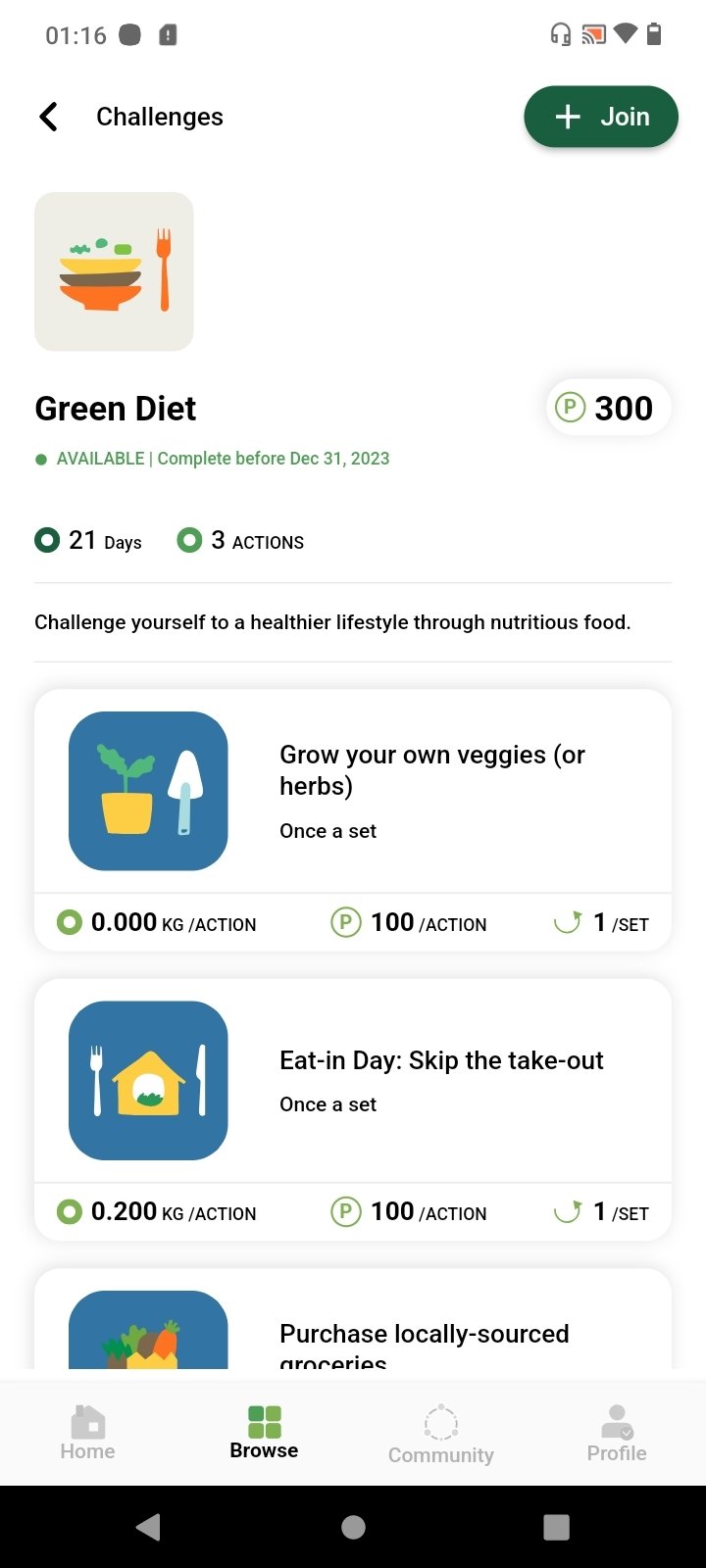Here is a cleaned-up, detailed caption for the image:

---

The image is a vertically-oriented screenshot taken from a smart device, against a white background that appears to be from a computer screen. At the top left corner, the time "1:16" is displayed, followed by a series of gray icons including a headphones icon, a filled triangle, and a battery life indicator. Below these icons, an arrow is pointing to the left next to the text "Challenges."

Beneath, there is a green button with a plus sign and the word "Join" in white text. To the left of this button, there is a picture featuring bowls and a fork, accompanied by the text "Green Diet." Adjacent to this, it states, "P300 available. Complete before December 31st, 2023" in green text.

Below, there is a rounded icon with "21 days, 3 actions" written inside it, emphasizing the challenge of adopting a healthier lifestyle through nutritious food. Under this section, there are several images with corresponding text and information:

1. "Grow your own veggies or herbs" – Each action saves "0.000 kg" and rewards "P100" per action with a 1% completion rate.
2. "Eat in, skip the takeout" – Saving "0.200 kg" per action, this action rewards "P100" for each set.
3. Partially visible text indicating "Purchase locally sourced groceries."

At the bottom of the screen, navigation options are displayed: "Home," "Browse" (which is currently selected), "Community," and "Profile." Alongside these options, the typical triangle, circle, and square buttons are visible on a black background.